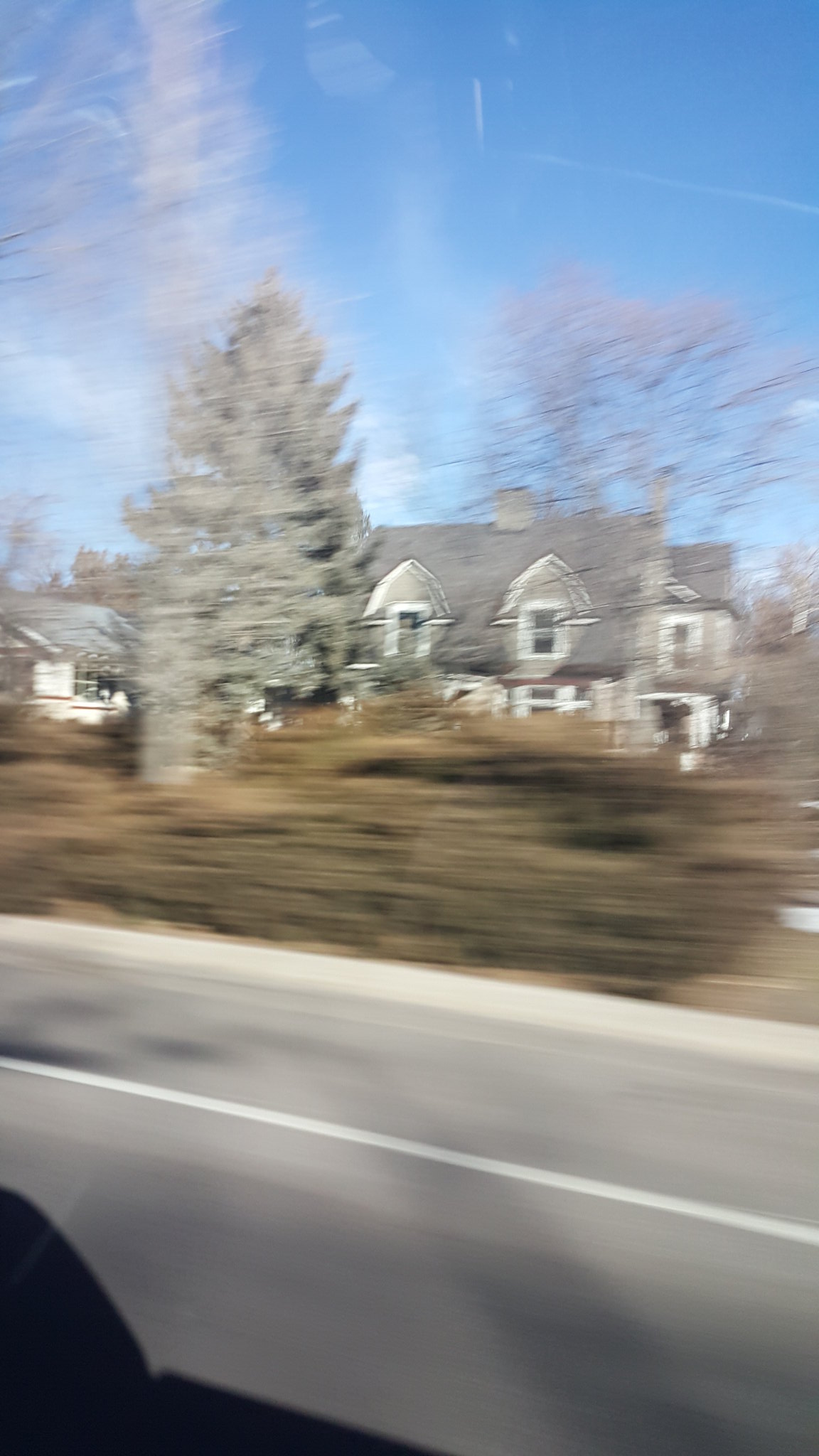The image captures a scene viewed from the passenger seat of a moving car, evident from the heavy motion blur and the partial view of a car window at the bottom edge. Dominating the foreground is a road marked with a white lane line, adjacent to a light gray sidewalk. A blurred green hedge runs alongside the road, partially obstructing the view of a two-story house. The house features light gray siding, numerous white-bordered windows, and a dark gray slanted roof with a chimney in the center. In the yard, to the left of the house, stands a tall, dark green pine tree that towers over the structure. Behind the house, a few sparse, nearly bare trees are visible. The backdrop includes a clear blue sky with a few wispy, swirling white clouds.